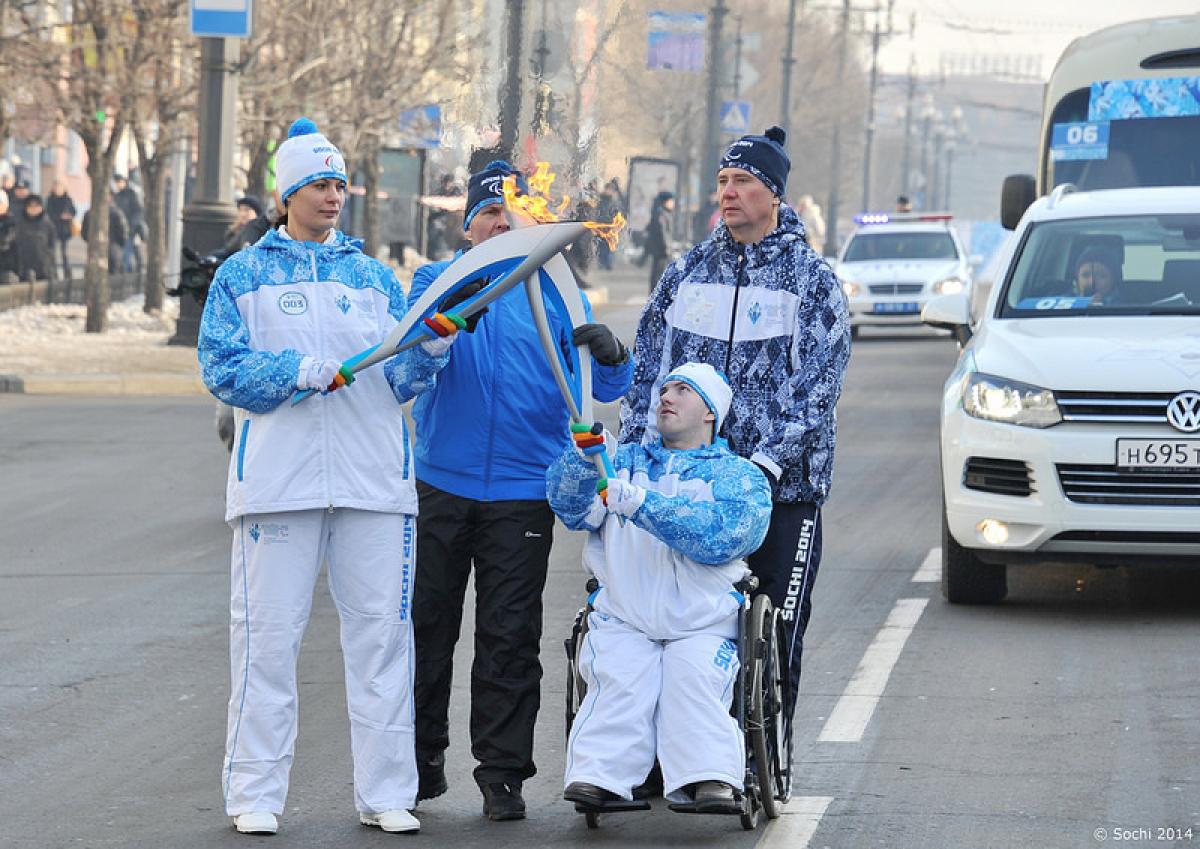The image depicts a winter scene on a city street, with four individuals prominently positioned in the foreground. To the left stands a woman in white athletic pants and a white-and-blue windbreaker jacket, donning a white winter hat with blue trim and a blue puffball. She holds a silver-and-blue curved torch. Next to her is a man in a blue windbreaker jacket, dark track pants, and a dark blue winter hat with a blue puffball. Another man stands to his right, wearing a blue-and-white windbreaker, dark athletic pants, and a dark blue winter hat. He stands behind a man in a wheelchair, who is dressed similarly to the woman on the left, in white pants, a white-and-blue windbreaker, and a matching winter hat. The man in the wheelchair holds another silver-and-blue torch, upright, transferring a flame to the woman's torch. In the background, a snowy roadside is visible, with bare trees and pedestrians on the sidewalk. Vehicles, including a white VW with a trailer and a police car with sirens, are positioned on the right. The scene suggests a ceremonial event, possibly related to the Olympic or Paralympic Games, as implied by the torch relay. Traffic appears stopped and a crowd of people seem to be watching the event.